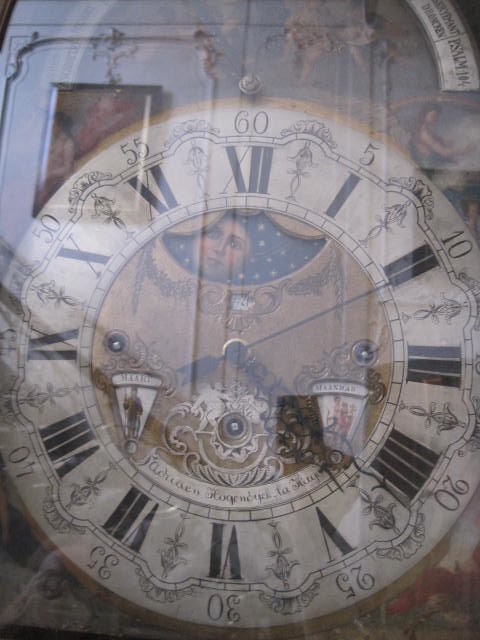The photograph captures a close-up of a uniquely designed, grand old-fashioned clock, possibly from the 1700s. The clock face, which dominates the frame, is cream-colored with black Roman numerals, each accompanied by smaller numerical digits like 5 and 10 over the 2, and 15 over the 3. Intricate, swirl-like designs, resembling skeleton motifs, embellish the spaces between the numerals. The clock also features a tan center surrounded by a grid-like stripe. At the top of the dial, there is a gold-plated cutout revealing a moon with a human face set against a starry blue sky. Below the hands, delicate writings can be seen. The clock appears to be slightly mirrored, reflecting an image of a picture hanging on a wall behind it. The photograph is somewhat blurry, making it challenging to distinguish if some images are part of the clock's reflections or inherent designs. Despite the blur, the clock's ornate and historical design stands out, emphasizing its beauty and uniqueness.